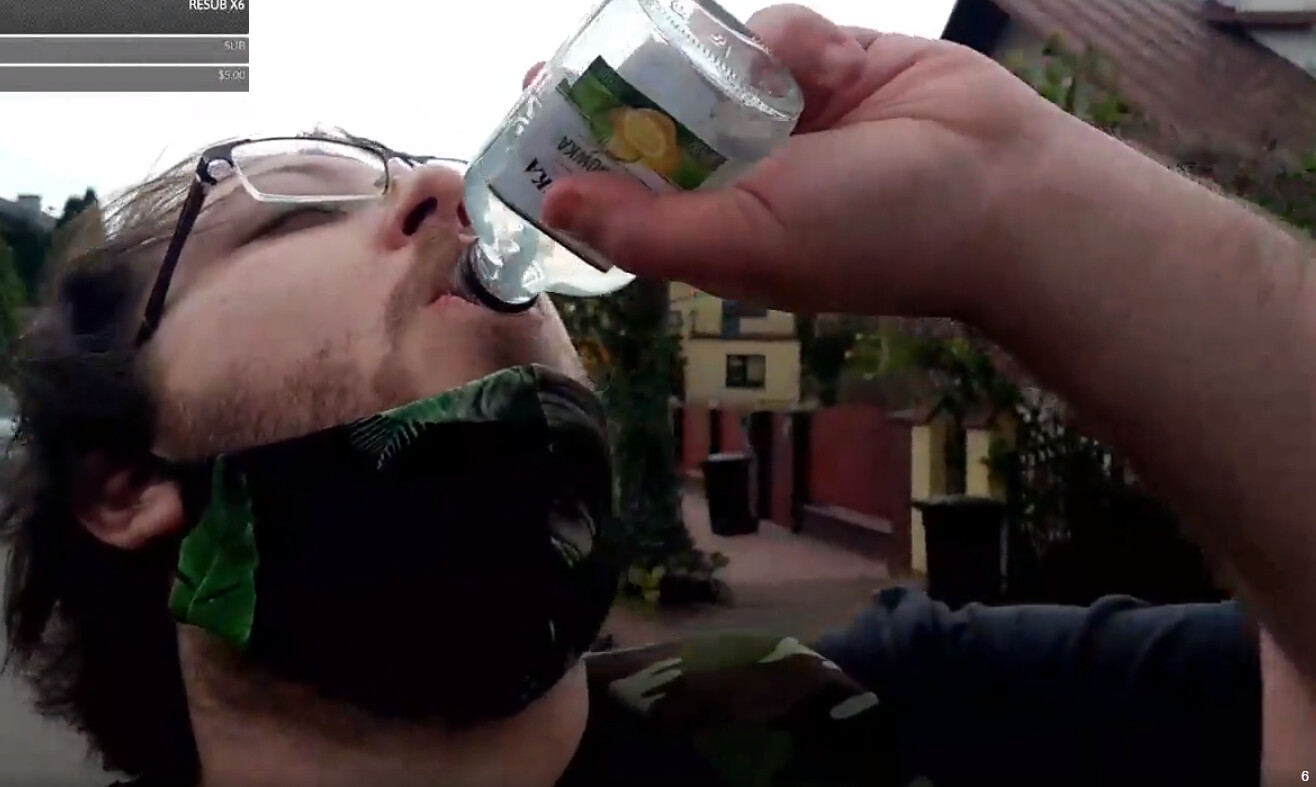This color photograph, taken outdoors during the daytime, features a close-up portrait of a gentleman drinking from a small, clear glass bottle of orange or lemon-flavored vodka, identifiable by the fruit illustrations on the label. The man is wearing a blue t-shirt and a camouflage backpack. His head is tilted back as he drinks from the bottle, which he holds up to his mouth. He wears black-framed glasses with clear lenses, and a black face mask decorated with green leaves is pulled down around his chin. His hair is dark brown and slightly short, and he has a sandy-colored, almost reddish beard and mustache. Behind him, a yellow house with a red-tiled roof and reddish-brown garage doors is visible, indicating the setting is in a residential area.